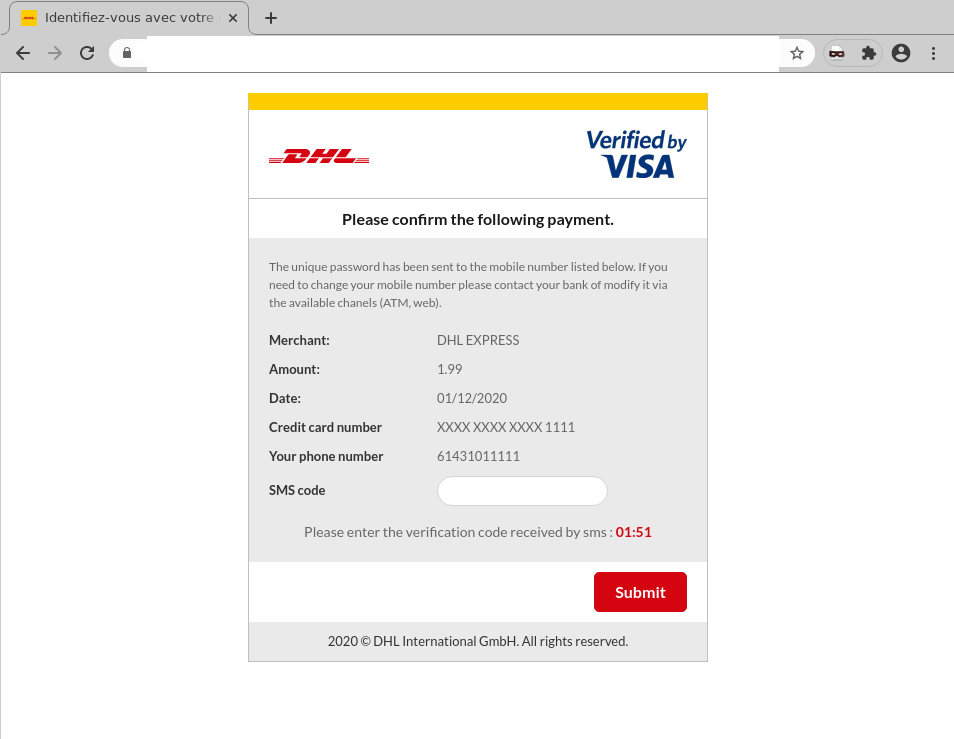A screenshot of a DHL payment verification webpage, which appears to be in French, is displayed. At the top, there are browser controls such as a gray tab with text reading " identifiez-vous avec votre" and options to exit the tab, add a new tab, navigate back, refresh the page, and perform a search. Additionally, an incognito mode icon is visible. 

Below these controls, a large dialog box features the red DHL logo on the left, and a blue "Verified by Visa" icon on the right. Following this, the text prompts the user to "Please confirm the following payment." A gray box provides details:

- Merchant: DHL Express
- Amount: $1.99
- Date: 01-12-2020
- Credit Card Number: **** 1111 (partial for privacy)
- Phone Number: 614-310-****

A field labeled "SMS code" is present with an empty input box for the user to enter the received code. Instructions advise entering the verification code received via SMS, for instance, "01-51," before clicking the red "Submit" button. At the bottom, the footer notes "2020 DHL International, all rights reserved."